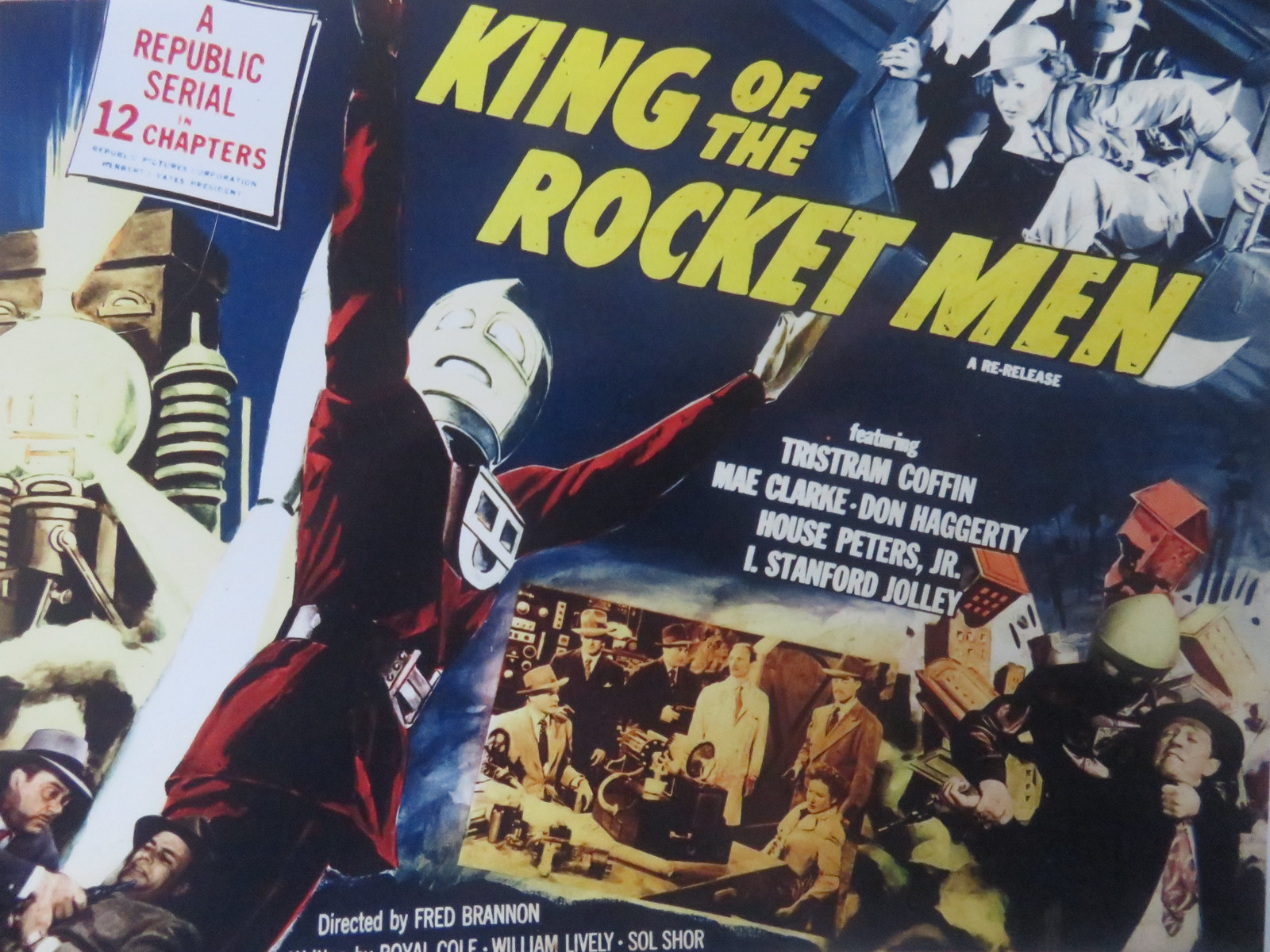This vintage movie poster advertises a re-release of the film "King of the Rocketmen." Dominating the center is an imposing figure clad in a red suit, complete with a thick belt and a silver, robotic mask. Their arms are dramatically stretched above them. Above this central figure, in bold yellow text, is the movie title: "King of the Rocketmen." The top left corner features a white text box with red letters stating, "A Republic Serial, 12 Chapters." Below the title, the poster lists the main cast: Tristam Coffin, May Clark, Don Haggerty, House Peters Jr., and L. Stanford Jolly. At the very bottom, it is noted that the film is directed by Fred Brannan.

Surrounding the central figure are various scenes and characters from the movie. On the left, there's an image of a man standing around a piece of vintage equipment. On the right, a scene shows a robot-like figure with its arm around a man's neck, the man sporting a hat. In the upper right corner, a woman wearing a hat appears to be in distress, seemingly trying to escape from something. This array of vivid details and dramatic poses creates a dynamic and intriguing advertisement, capturing the essence of the serial's adventurous spirit.